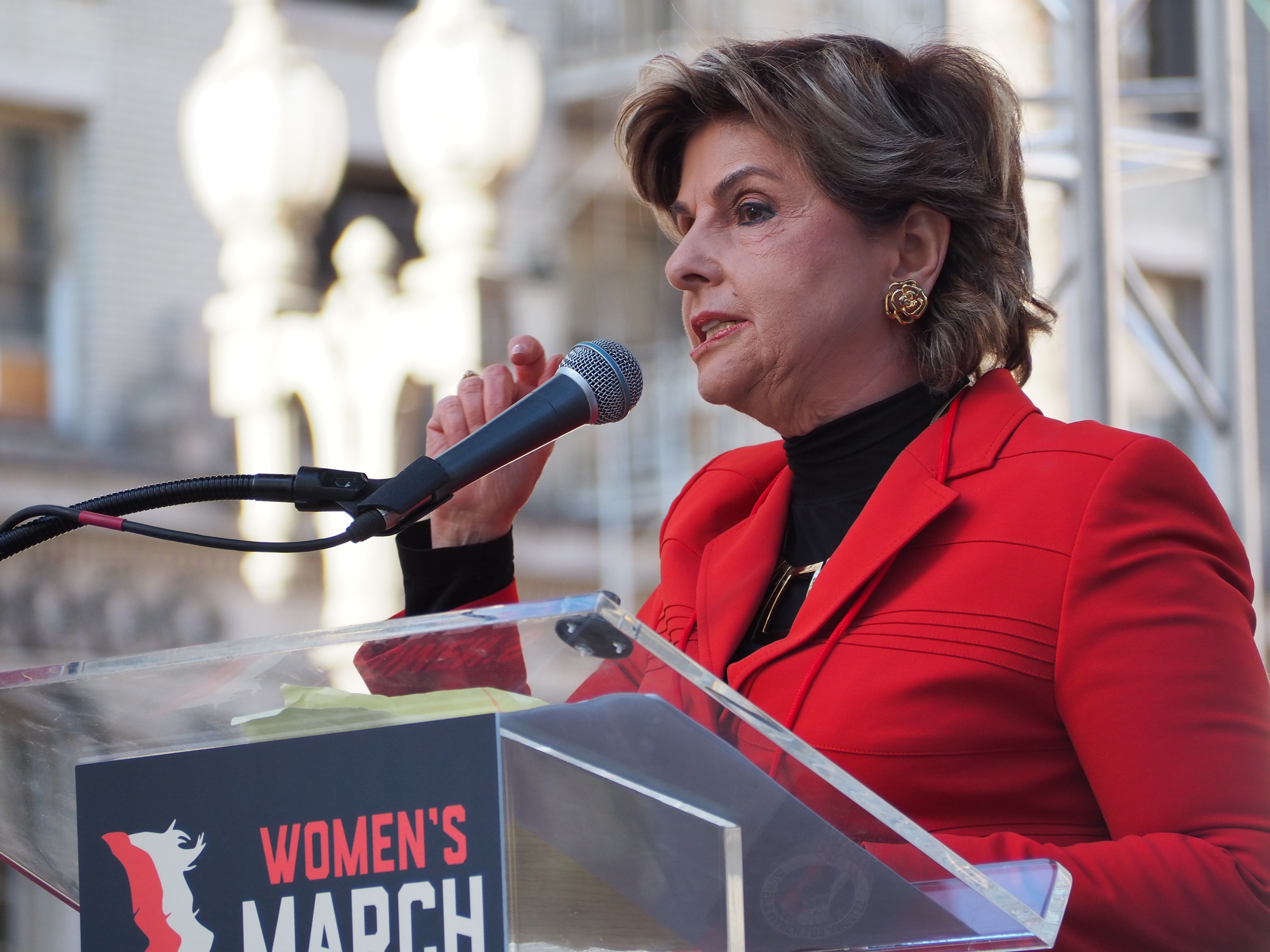The color photograph captures a woman, who closely resembles lawyer Gloria Allred, standing at a clear, see-through plastic podium adorned with a sign that reads "Women's March" in red and white letters alongside a red and white logo. She has a light skin complexion and short brown hair with gray or blonde streaks, and she wears round gold earrings on her visible left ear. Dressed in a red suit jacket over a black turtleneck, she accessorizes with a partially visible gold necklace. The woman is in mid-speech, facing slightly to the left with her mouth open and her right arm raised, her hand near a black and silver microphone positioned directly in front of her face. The backdrop includes a streetlamp and a stone or brick building with windows, indicating an outdoor setting. The scene is well-lit, highlighting the clarity and details of the moment.